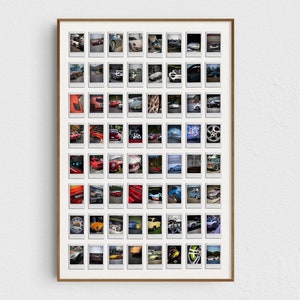Mounted on a stark white wall is a framed poster featuring a thin gold frame and a white mat. The poster itself displays a grid of 64 tiny rectangles, arranged meticulously into 8 columns and 8 rows. Visible in these small rectangles are Polaroid photos, each retaining the classic Polaroid format with a white margin at the bottom. Although the individual photos are too small to discern clearly, their collective arrangement is suggestive of images, possibly cars based on a closer look. The overall image is clear, set within a bright, naturally-lit environment which accentuates the details of the grid and frame.